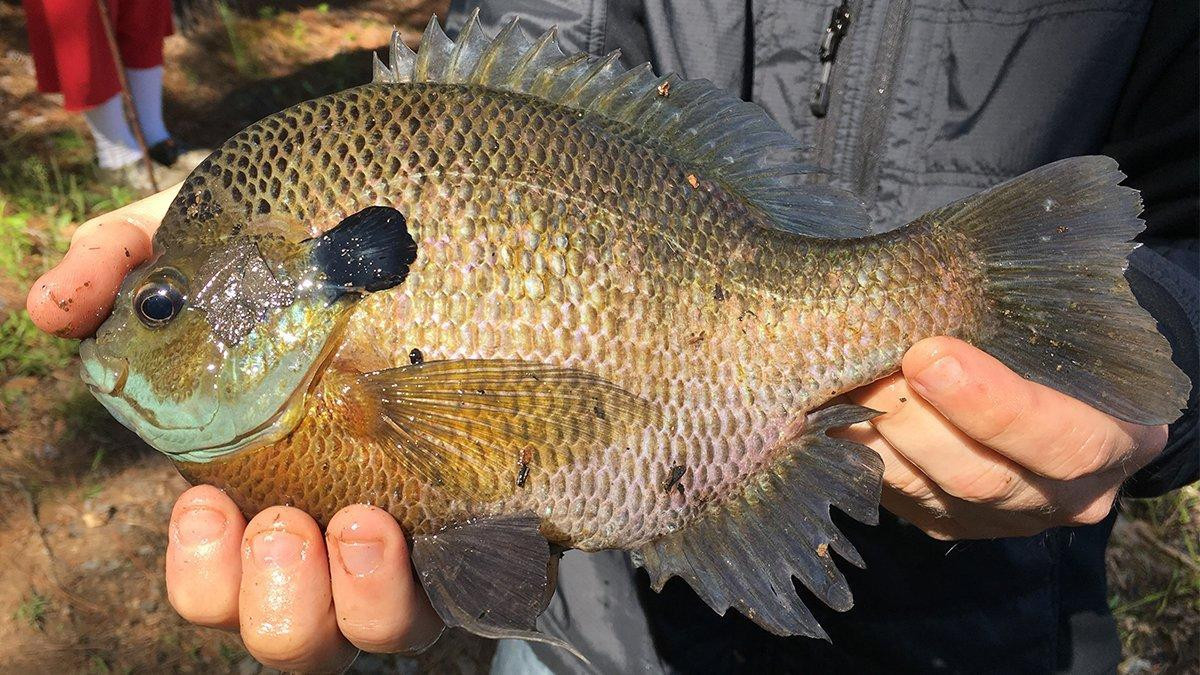In this detailed photograph, a fish is being held by a person whose hands are visibly dirty with sand and mud. The person, cropped out at the head and torso, is wearing a black or bluish zip-up jacket. The background includes grass, dirt, and the partial view of another individual in white socks, a red dress, and holding a wooden cane, suggesting an outdoor setting on a sunny day.

The fish itself is relatively fat and not particularly long, approximately one foot in size, indicating a shorter and broader body shape akin to that of a flounder rather than the more torpedo-shaped bass. The fish's body is covered in numerous scales that display a symphony of colors: yellow-orange along the bottom, grayish underbelly, and darker shades of black and gray on top, with some hints of brown and shiny dark green across the scales. The fish features spiky, iridescent fins running from the middle of its back down to near its tail, as well as a longer bottom fin. Its eyes are black, and it has a slightly green hue around the cheeks and jaw area. The person is holding the fish with a thumb on its nose, three fingers under its head, and three fingers supporting its tail, indicating a careful grip due to the sharp spikes on its back. The sunlight reflecting off the fish’s scales adds a glistening, almost iridescent quality to its appearance.